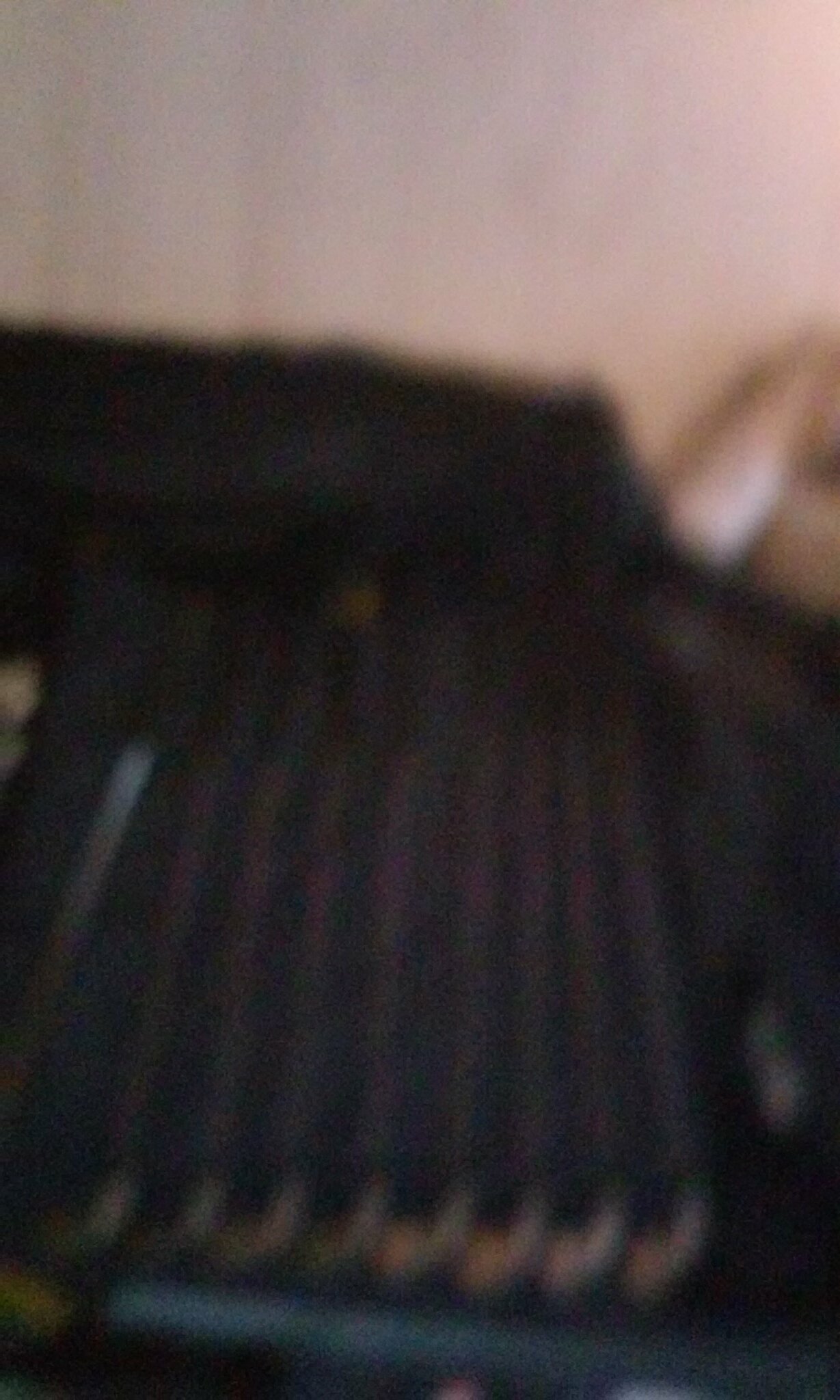The image depicts a partially blurred, close-up section of what appears to be a typewriter. The object is primarily bluish in color, with the edges and keys faintly visible despite the blur. The keys sit slightly below the formed back and sides of the machine. The background features a cream-colored wall, and behind the typewriter, there are indistinguishable, blurred objects, also in a cream hue with some black elements on top, all of which are equal in height. The overall composition suggests a vintage setting.